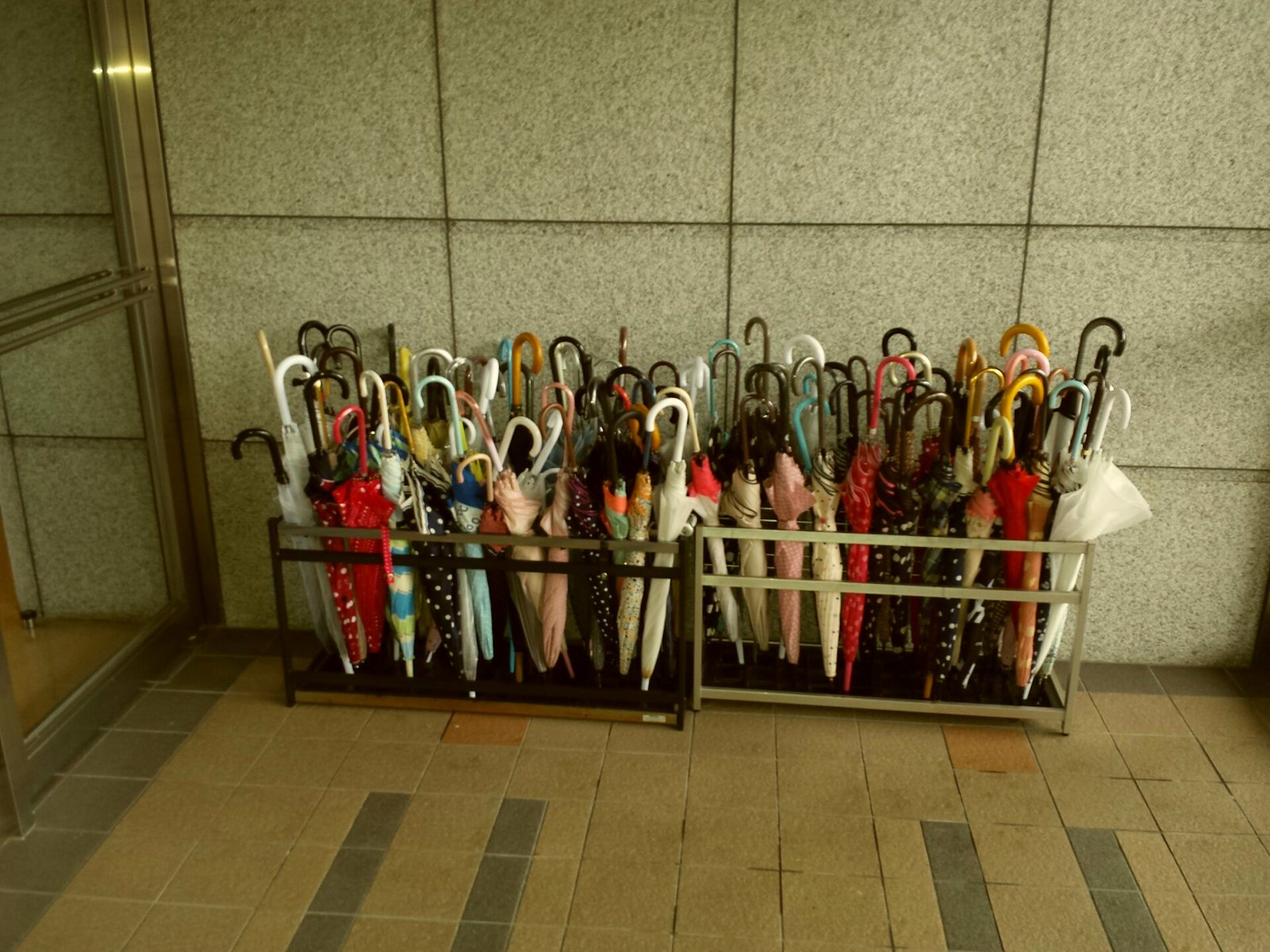This image appears to be a scene within a building, potentially a public space like a library or office, featuring a well-organized umbrella storage area. Dominating the scene are two grey racks filled with approximately thirty umbrellas each, displaying a spectrum of colors and patterns, from solid hues like white, black, yellow, and orange to various polka-dotted designs in red, black, and blue. The umbrellas are neatly placed with their handles up, ready for retrieval. The backdrop consists of a wall tiled with light grey stone squares arranged in a 4x3 grid, lending an orderly appearance to the space. The floor beneath is a mosaic of earth-toned tiles, interspersed with grey and orange, bordered by a grey trim. To the left side of the image, a greyish metal door frame for a glass door is visible, with two horizontal metal bars that seem gold in some descriptions, suggesting a refined touch. This meticulous setup hints at a high-traffic area where trust plays a crucial role, likely placing the scene in a context where community respect and the honor system are vital, possibly in Japan.